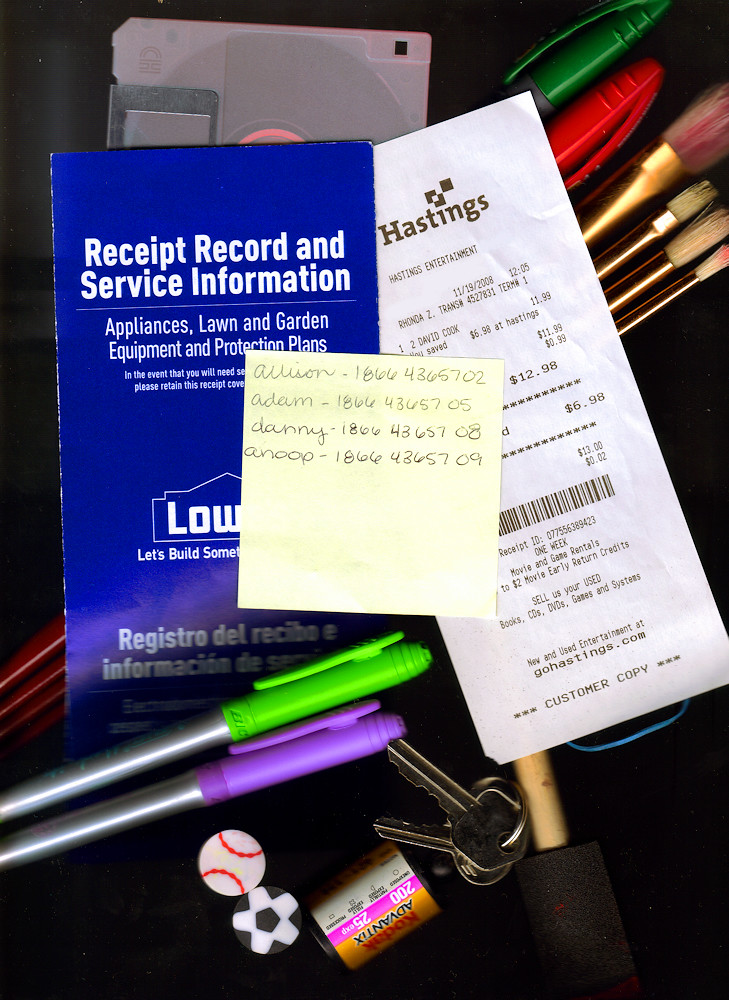A detailed and well-composed color photograph showcases a meticulously arranged assortment of items against a black background, giving the impression of a product collage. From top to bottom and layer by layer, the photo reveals various objects thoughtfully stacked and juxtaposed.

At the base of the composition lie four paint brushes of diverse sizes—the largest one placed prominently beside three smaller brushes, each distinct in their form and bristle pattern. Adjacent to these brushes, two pins capture the eye: one with a green tip and the other topped with red.

Further upward, a vintage 3.5-inch gray floppy disk provides a nostalgic focal point. Resting atop this relic are two paper receipts—the first from Hastings, itemized at $6.98, and the second a registration document titled "Received Record and Service Information." Crowning these documents is a post-it note, annotated with phone numbers for individuals named Allison, Adam, Danny, and Anoop.

Continuing the visual journey, two more pins are discovered below, bearing green and purple tops respectively. Nearby, a set of keys accompanies a small film canister—which may alternatively function as a quirky keychain—adding an intriguing touch to the narrative captured in this image.

This intricate assembly, artfully chronicled, invites the viewer to ponder the stories behind each item, blending memories and functionality within a single frame.